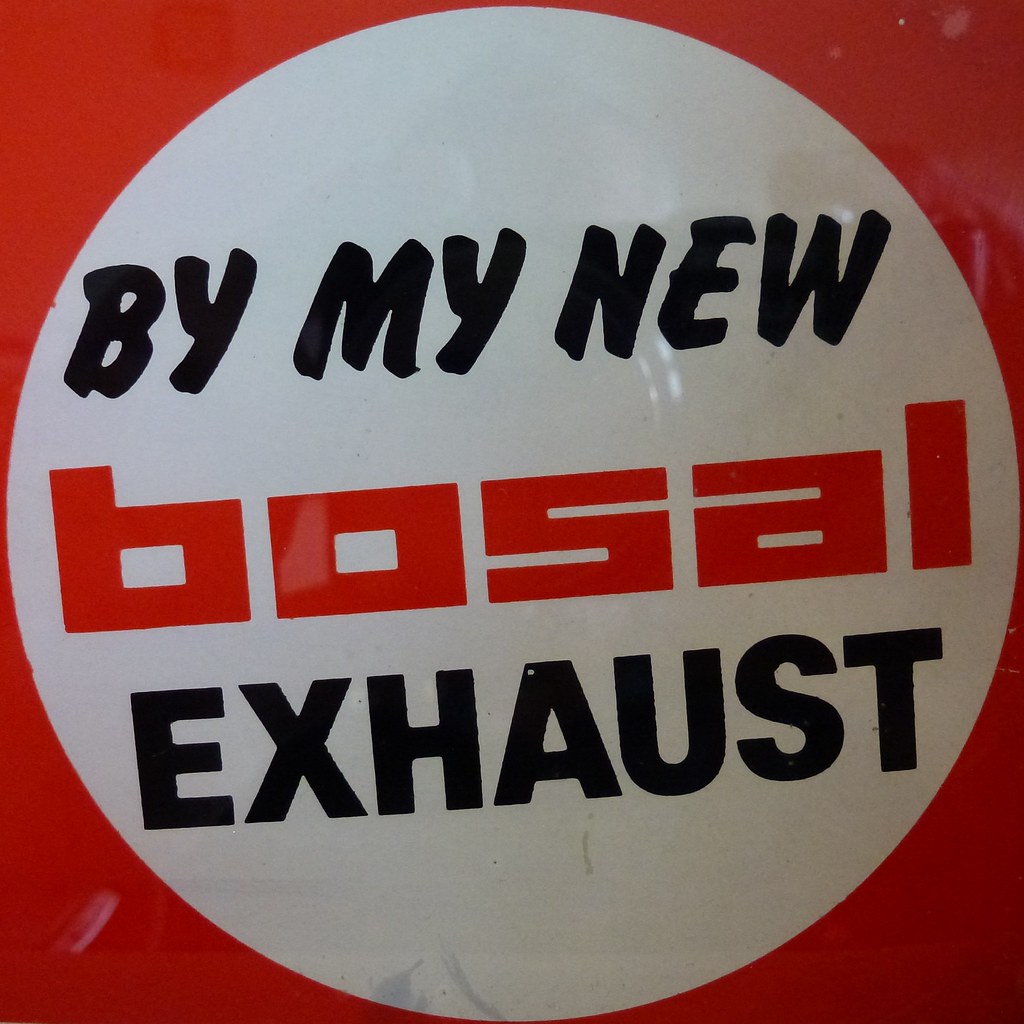The image features a vibrant red background with two distinct red triangles in the upper corners. At the center of this background is a prominent white, circular shape. Inside the circle, at the top, there is bold black text that reads "Buy My New" (B-Y space M-Y space N-E-W), followed by the word "BOSAL" (B-O-S-A-L) in red letters directly below. Underneath "BOSAL", the word "EXHAUST" (E-X-H-A-U-S-T) is displayed in bold, uppercase black letters. There appears to be a shiny effect on the image suggesting reflections or faded objects in the background, but the details of these are unclear. The only colors present in the image are black, white, and red, creating a striking visual advertisement for what seems to be an exhaust product from a brand named BOSAL.